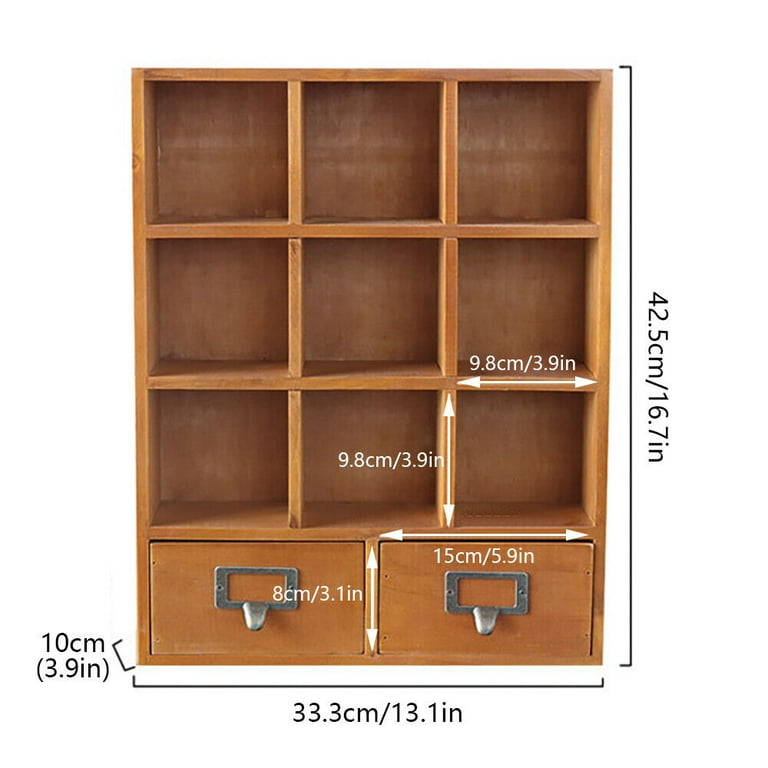The image depicts a wooden organizational unit designed for a desk, characterized by a light walnut color and compact structure. The unit features three rows of three cube compartments, making a total of nine, each measuring 9.8 centimeters (3.9 inches) in both height and width. Below these cubbies are two library-style drawer pulls, silver in color, resembling those found on library card catalog drawers. These drawers measure 8 centimeters (3.1 inches) in height and 15 centimeters (5.9 inches) in length. The overall dimensions of the unit are marked by black measurement lines: 42.5 centimeters (16.7 inches) in height on the right-hand side and 10 centimeters (3.9 inches) across the bottom width. White lettering within the image annotates the size of each cubby, ensuring the dimensions are clear.